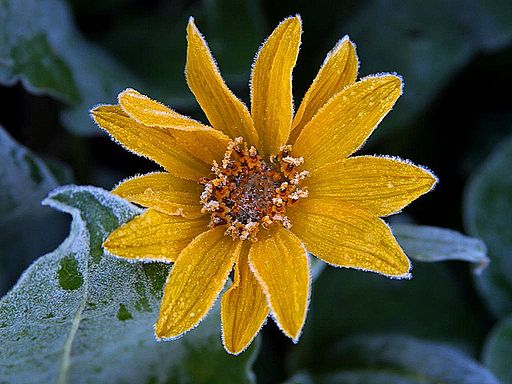This close-up photograph captures a dark yellow flower, possibly a gold leaf flower, after a light frost. The blossom, positioned centrally, features approximately 15 oval-shaped petals arranged in two slightly overlapping rows. Each petal is illuminated with specks of white, suggesting a dusting of snow or possibly a frost. At the flower's core, tiny stems transition from orange near the base to white at the tips, encircling a center displaying copper and brownish hues. Surrounding this striking bloom, the leaves are detailed with a subtle white substance, hinting at either frost or pollen, adding texture and depth to the image.